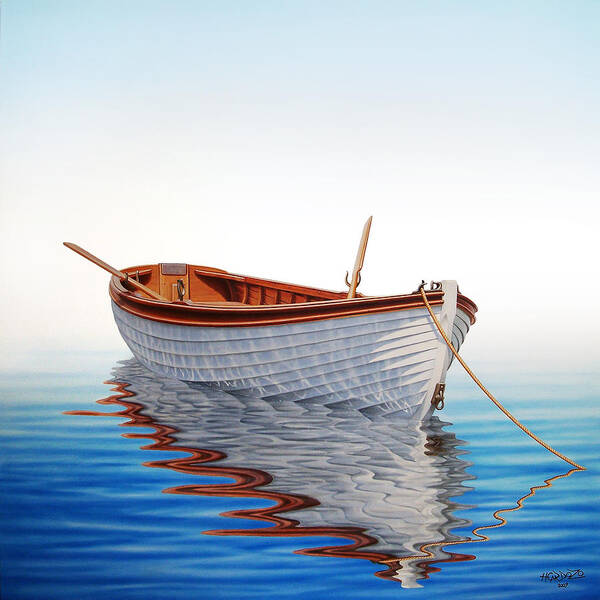This is a detailed painting of a small white wooden rowboat with a stained wooden interior and brown trim, anchored in a body of water. The boat has two wooden oars, one on either side, sticking up from the inside. A long rope leads from the bow of the boat into the water, ending with a brass hook near the water's edge. The reflection of the rowboat is visible in the water, but it is dramatically rippled, giving the effect as if the boat is melting. The sky is a bluish gray with no detail, suggesting an overcast afternoon. Ripples on the water surface further distort the reflection of the boat, adding a sense of movement and fluidity to the otherwise still scene. The painting is signed, although the signature is not clearly legible.